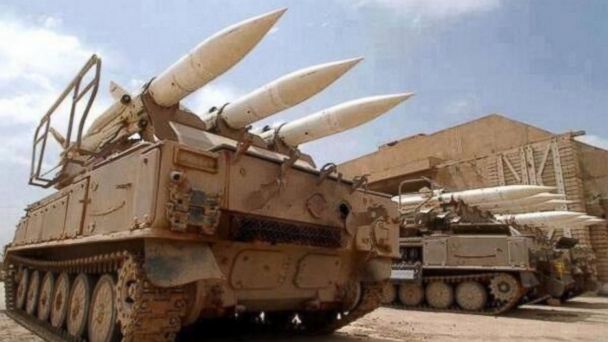In this photograph, we see an arrangement of three beige-colored tanks, each equipped with three white missiles that are small, thin, and pointed at the ends. The foreground is dominated by a large tank, nearly filling the viewer's vision, with two additional tanks lined up beside it. Despite the traditional treads and wheels common to tanks, these vehicles lack elongated gun barrels, suggesting they function as missile carriers rather than standard combat tanks. All three tanks are stationary, set in a sunny, desert-like environment with dusty ground that hints at the Middle East. Light clouds dot the mostly clear sky, and the bright sunlight casts distinct shadows of the tanks on the ground. In the background, there's a cement bunker with a large garage door, likely the tanks’ origin.